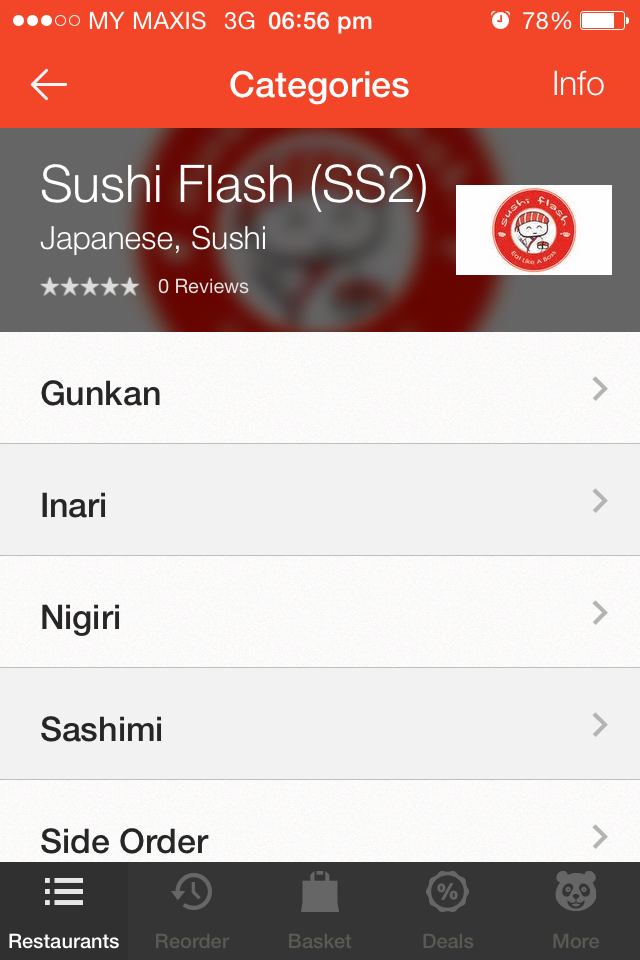This image captures a screenshot from a mobile phone displaying the Sushi Flash SS2 section under the category 'Japanese Sushi' on a food ordering app. The interface shows that the establishment currently has zero reviews, accompanied by a five-star rating system that remains uncolored. The header of the page is a striking red hue with navigation options, including 'categories' at the top, a left-pointing arrow icon for navigation on the left, and 'info' on the right. 

Below the header, the app's interface transitions to a gray background featuring a list of sushi categories: 'Gun Can,' 'Inari,' 'Nigiri,' 'Sashimi' (spelled 'S-A-S-H-I-M-I'), and 'side order.' The bottom section of the screen is lit up within the gray background and showcases a black rectangular menu with various options: 'restaurants,' 'reorder,' 'basket,' 'deals,' and a 'more' option highlighted by a panda bear's face above it. The overall layout succinctly organizes sushi options and provides navigational ease for users.